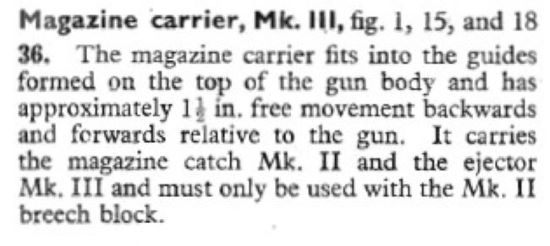The image appears to be a black and white text snippet extracted from an old newspaper or magazine. The layout consists entirely of text positioned centrally on the white background, with certain phrases emphasized in bold. At the top, the bolded text reads "Magazine Carrier MK3, Figure 1, 15, and 18, 36." The detailed description within the text explains that the "magazine carrier fits into the guides formed on the top of the gun body and has approximately one and a half inches of free movement backwards and forwards relative to the gun." It further notes that the carrier holds the magazine catch (MK2) and the ejector (MK3), and specifies that it must be used exclusively with the MK2 breech block.